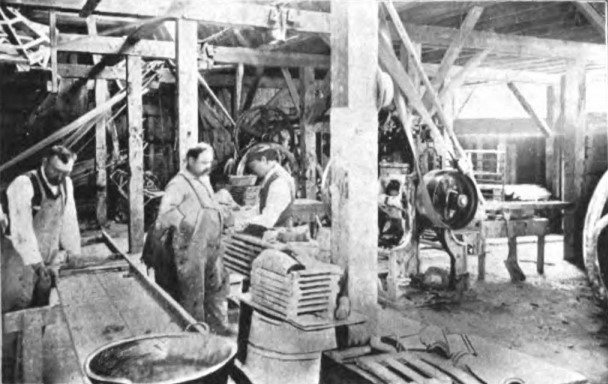A black and white photograph captures the interior of an old factory with wooden beams supporting both the ceiling and walls. The large room, suffused with natural light from a window in the upper right corner, features a mixture of machinery and workspaces. On the right side of the image, a large machine with a prominent wheel and drive belts stands near several men wearing overalls and long-sleeved shirts. One man, identified by his dark hair and suspenders, appears to be holding an object, while the others observe. To the left, a long wooden table stretches into the distance with a man leaning over it, presumably engaged in a task, possibly sanding wood or bending something. In the foreground, a large metal bowl and other miscellaneous objects, such as a pallet, add to the cluttered, industrious atmosphere. The men, who all seem to be Caucasian with fairly light skin, are captured in various stages of work and interaction, embodying a sense of simple, earnest labor.